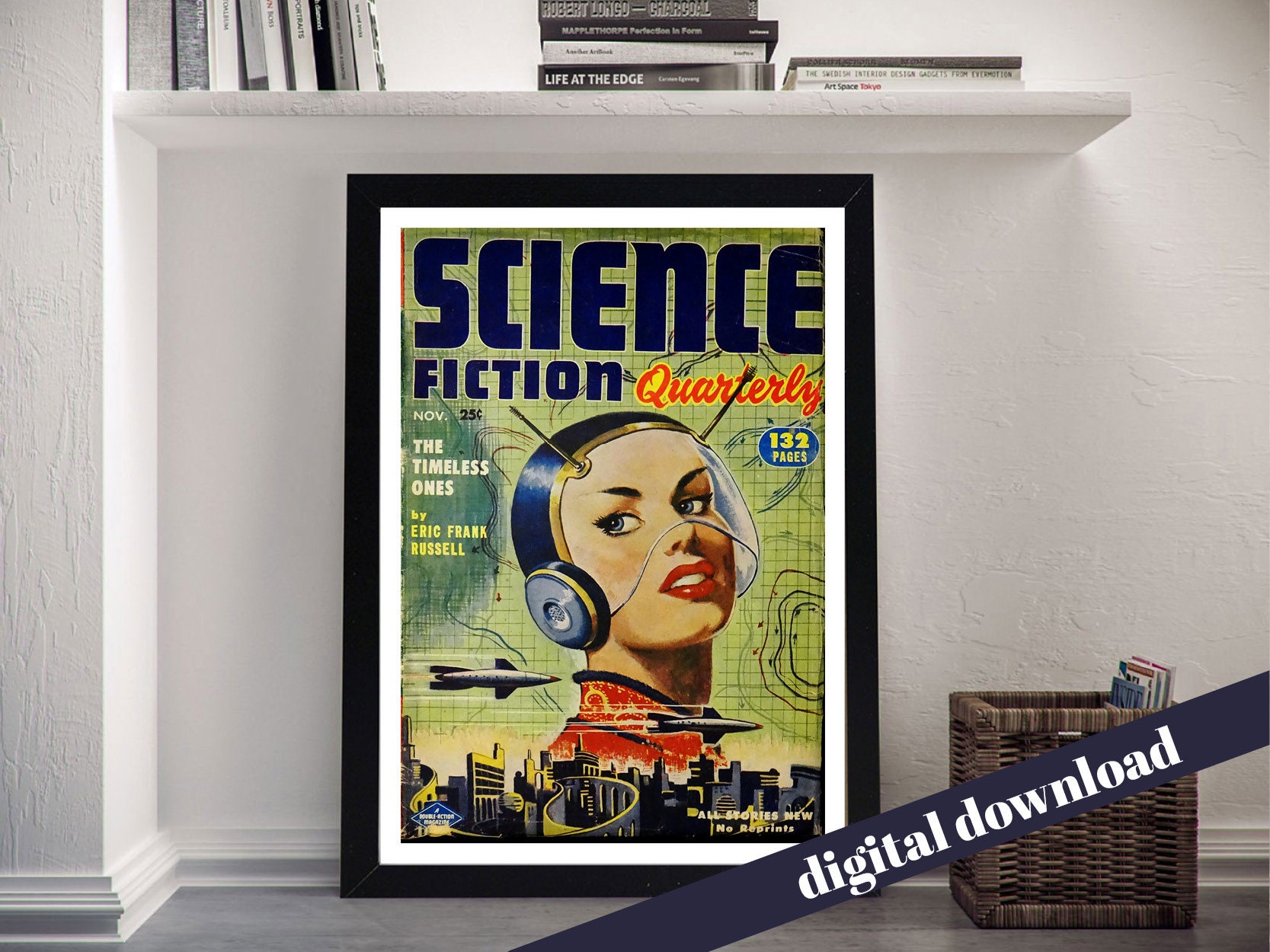The image depicts a meticulously arranged modern room with white walls and a gray floor, complemented by a wooden border at the base. Prominently displayed against the white backdrop is a large, framed poster titled "Science Fiction Quarterly". The title features "science fiction" in striking blue letters and "quarterly" in red. The cover portrays a futuristic drawing of a woman donning a blue and gold helmet with a glass visor, obscuring her hair. Two antennas protrude from her forehead, reminiscent of an insect's feelers. Her visage is adorned with red lipstick and subtle eye shadow, and she wears a red, perhaps culturally inspired, turtleneck outfit. Below her neck, a stylized skyline of yellowish, black, and dark blue buildings is depicted, with planes flying overhead. 

To the left of the frame, text indicates "November NOV" and "25 cents", followed by "The Timeless Ones" by Eric Frank Russell. The right side notes "132 pages" and details that all stories are new, with no reprints. The background of the poster is green with intricate black outlines and lines, akin to a technical diagram. 

A simple, white shelf at the top holds a variety of books, including "Life at the Edge," "Robert Longo," and "Charcoal", alongside a stack of magazines in a nearby wicker basket on the floor. The presence of a banner in the bottom right corner of the image reading "digital download" hints at the possibility of the image being used for advertising or purchasing purposes.